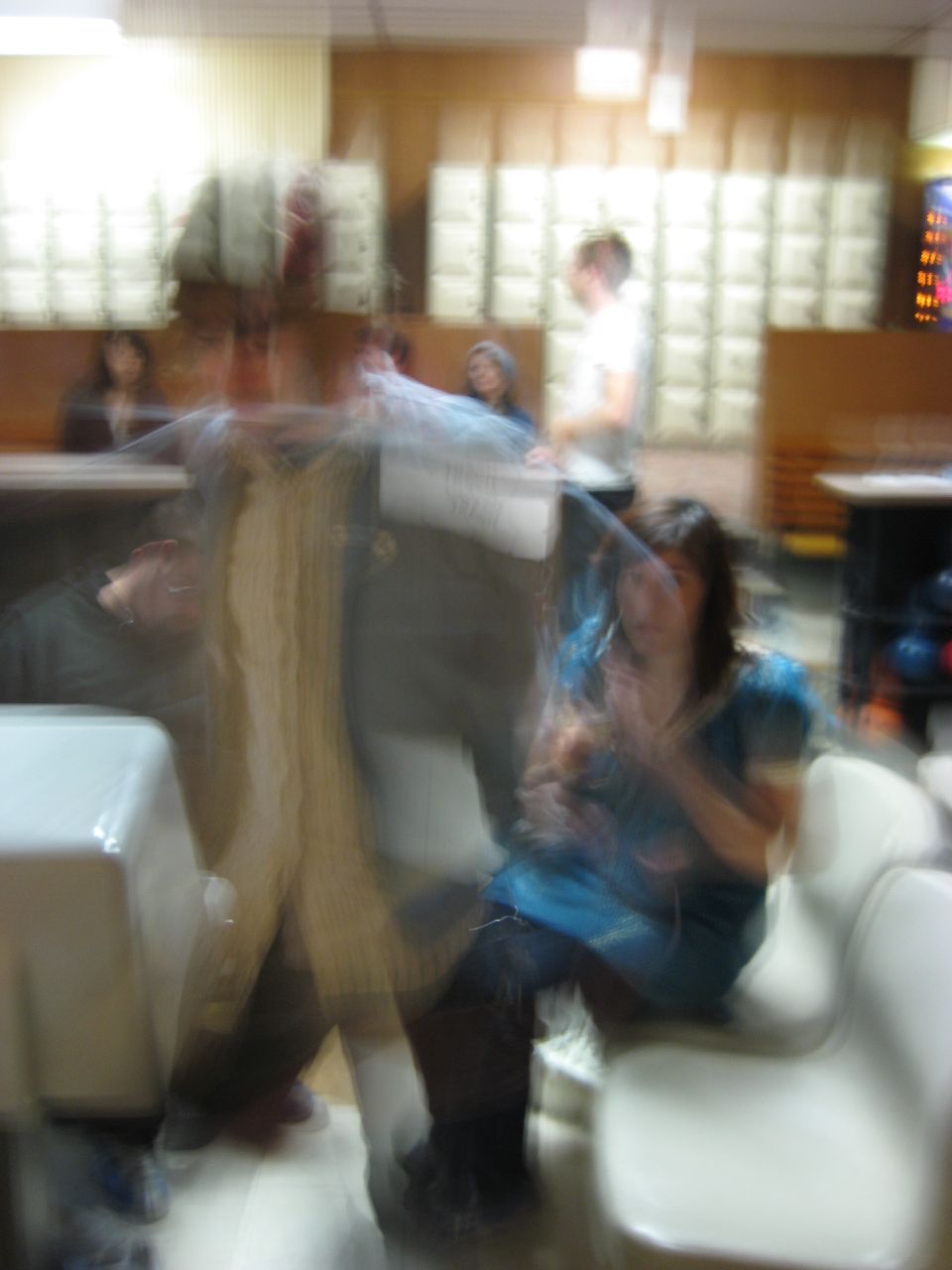In this blurry, portrait-oriented image, the main focus is a woman seated on an upholstered white chair within an office environment. She has long, straight black hair and appears to be Caucasian. She is dressed in a blue blouse and black pants. The setting includes another man standing at the end of a table behind her, with a slightly obscured group of at least two women seated along the same table. There appears to be something indiscernible between the two women, possibly hiding a third figure. In the background, the room is well-lit due to ceiling-to-floor windows that extend above a half-wall, allowing natural light to flood the space. The man is positioned in front of an opening in this half-wall, and to the viewer's right, the wall continues seamlessly.